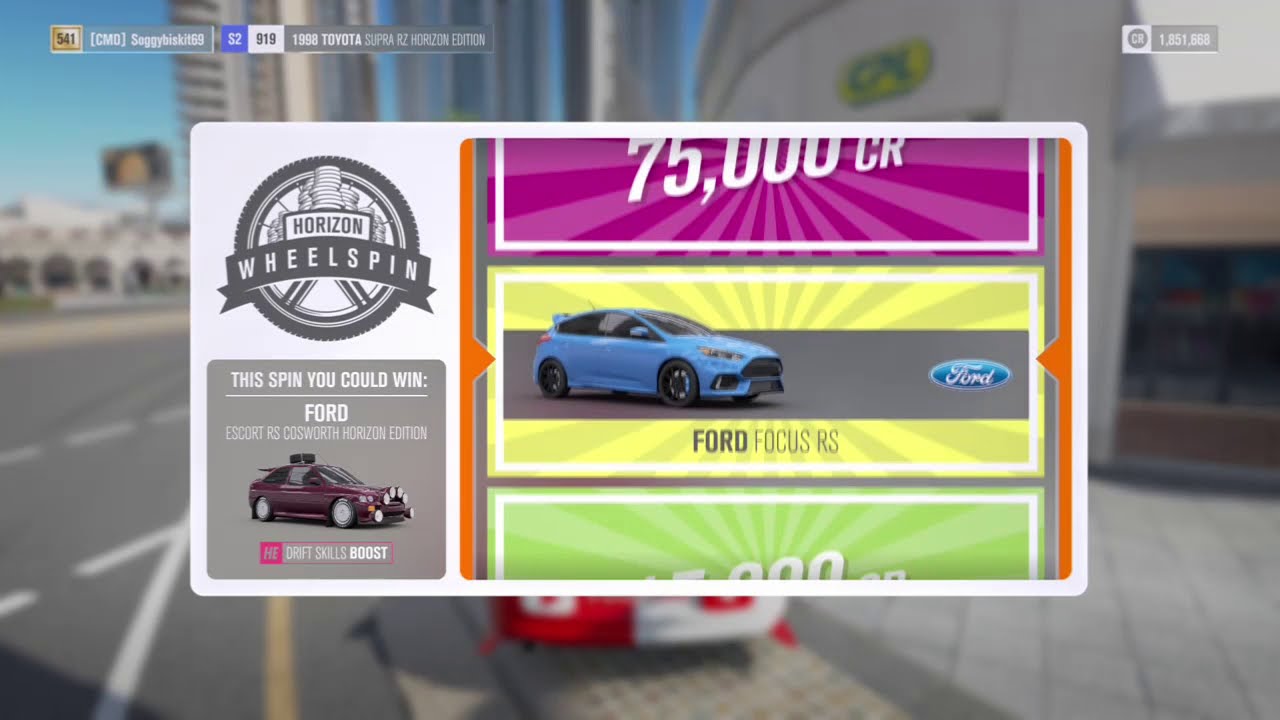This is a highly detailed screenshot from a sophisticated video game, depicting a pop-up advertisement for a "Horizon Wheelspin." Dominating the center of the image is a circular wheel or tire icon, emblazoned with the text "Horizon Wheelspin" across a banner. The upper left contains an icon that looks like a tire with the words "Horizon Wheelspin" in black and white, overlaid with a banner that resembles piles of gold coins.

Below this, a gray square displays the message, "This Spin Could Win," followed by "Ford Escort RS Cosworth Horizon Edition," indicating a prize vehicle. The showcased car is a souped-up, red Ford Escort RS Cosworth Horizon Edition, visible from the passenger side, featuring multiple headlights, a dark-tinted window, a rear spoiler, and what appears to be a tire strapped to the roof. The car offers a "Drift Skills Boost" as noted beneath the vehicle.

To the right of the pop-up, the ongoing wheelspin is framed by two orange lines and currently highlights a "Ford Focus RS" panel. This section shows a blue Ford Focus against a yellow background, accompanied by the Ford logo and the text "75,000 CR," suggesting an in-game currency reward. The entire scene is set against a backdrop of city buildings and roadways, enhancing the ambiance of this immersive video game environment.